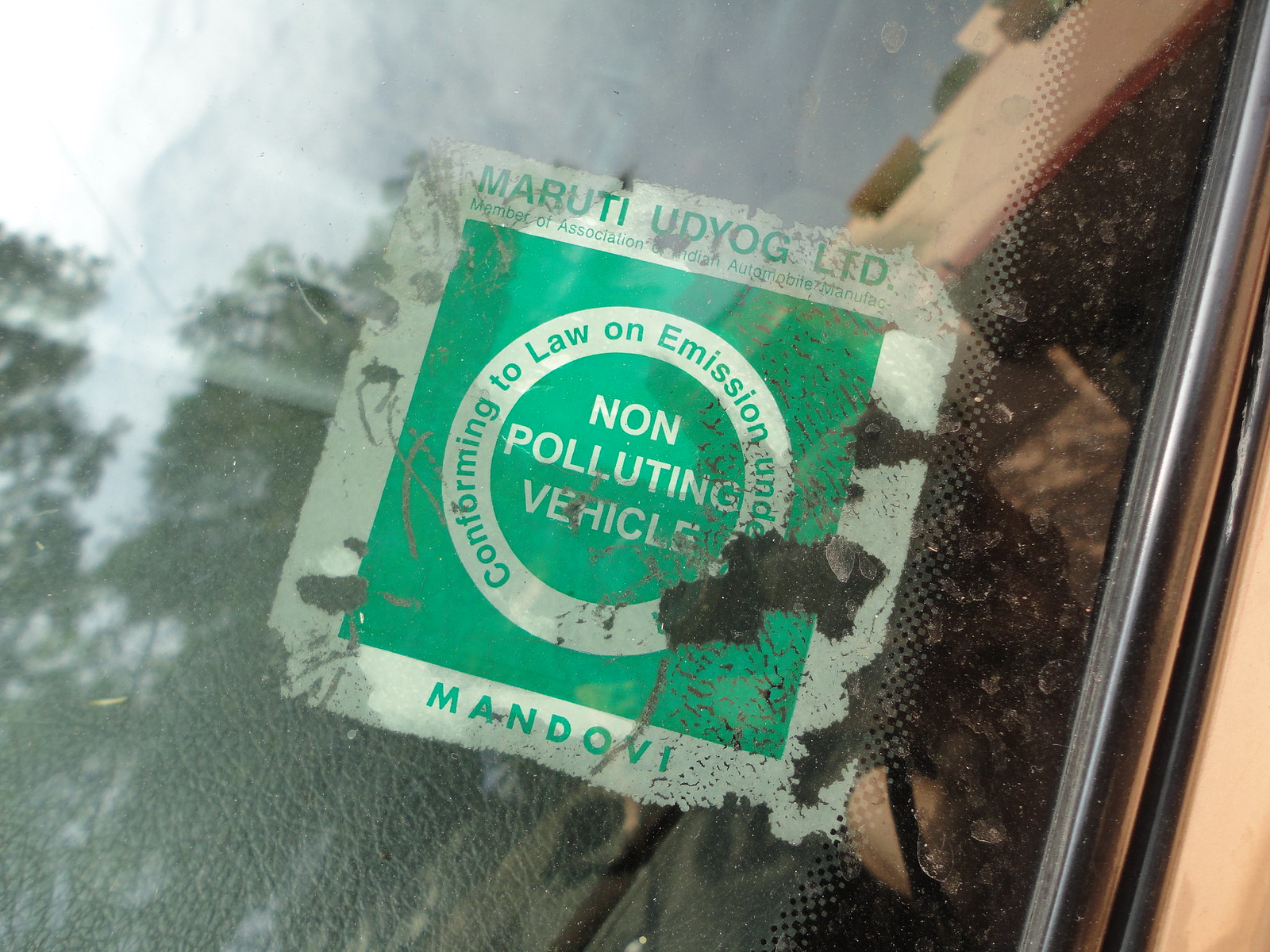This is a color photograph taken outdoors of an old regulation sticker affixed to the windshield of a car, reflecting trees in the background. The windshield belongs to a car painted in a copper or chrome color. The sticker is square and features a white background with green text and elements. At the top, it reads "Maruti Udyog Limited," identifying it as part of the Indian Automobile Association. Below this, in a clear green triangle, it states "Conforming to Law on Emission, Non-Polluting Vehicle." At the bottom of the sticker, the word "Mandovi" is prominently displayed in all capital letters: "M-A-N-D-O-V-I." The sticker, which is marked with gouges and grime, gives the impression of considerable age but remains legible.